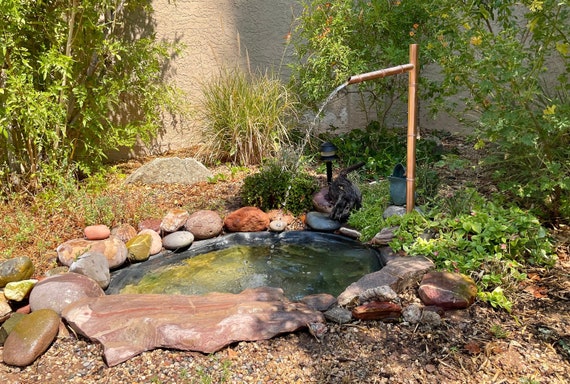This color photograph features a quaint, man-made fountain set in a small, serene pond surrounded by a charming landscape. The pond, free of fish, showcases clear water and is lined with a variety of uniquely shaped and colored rocks, including rounded river rocks and angular stones in hues of red, gray, and white. Emerging from the center, a simple yet elegant brass-colored, copper pipe arches water gently into the pond, which appears to be supported by a wooden stake. The scene is framed by lush green plants and shrubs, enhancing the natural beauty of the feature. A stucco wall forms the backdrop, adding a touch of rustic charm to the peaceful setting. Notably absent from this tranquil image are people, animals, buildings, and vehicles, focusing the viewer's attention solely on the harmonious garden oasis.